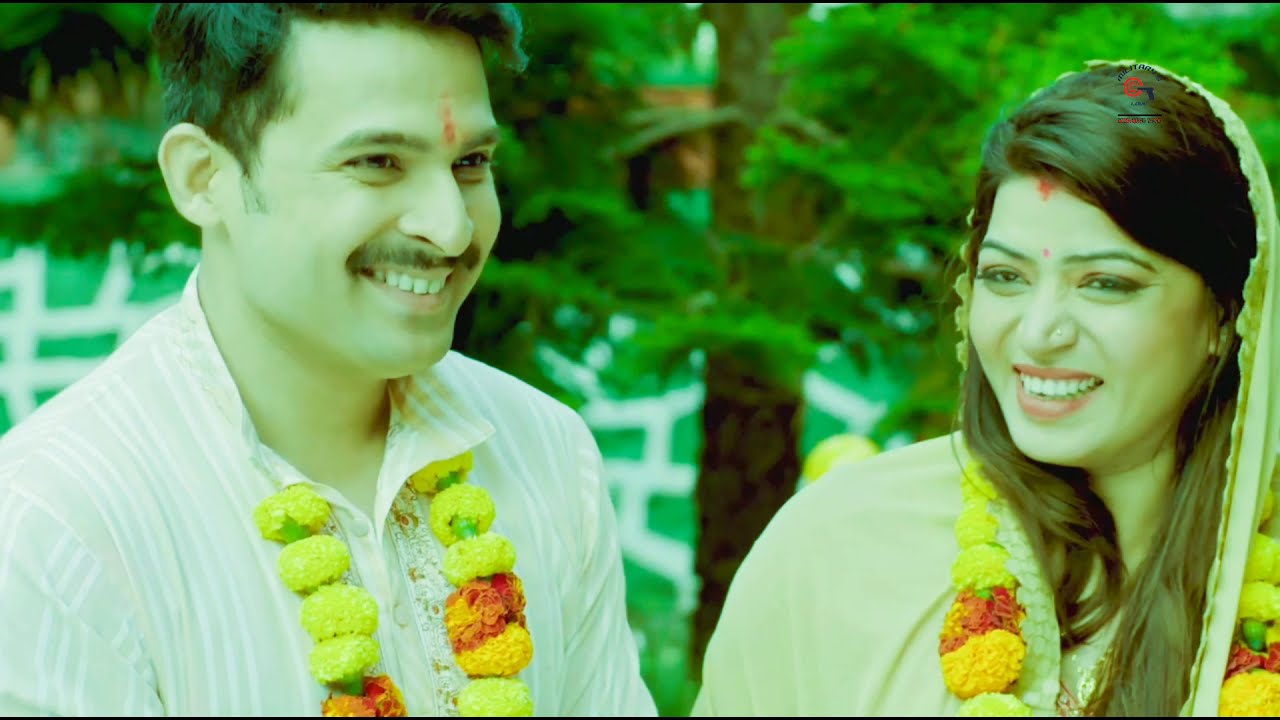This photograph captures a joyous moment likely from an Indian wedding or celebration. It features two individuals of possibly Indian or Arab descent, with the male on the left and the female on the right. Both are adorned with elaborate flower necklaces, predominantly featuring yellow and orange marigolds, indicating a festive occasion. The man, smiling warmly, has a short brown hairstyle and a thin black mustache, and is dressed in a white, vertically striped collared shirt, unbuttoned at the top. He also sports a traditional red mark on his forehead, common in religious or celebratory contexts.

The woman, also smiling, has long, dark brown hair and wears a beige outfit accompanied by a headdress. She, too, has a red mark on her forehead, along with makeup that highlights her pink lips. Her attire appears elegant and complements the ceremonial theme. A lush green tree, possibly a pine, stands behind them, adding a natural backdrop to the scene. The outdoor setting, coupled with their attire and accessories, suggests this image was taken during a significant cultural or religious event, marking a moment of happiness and celebration.